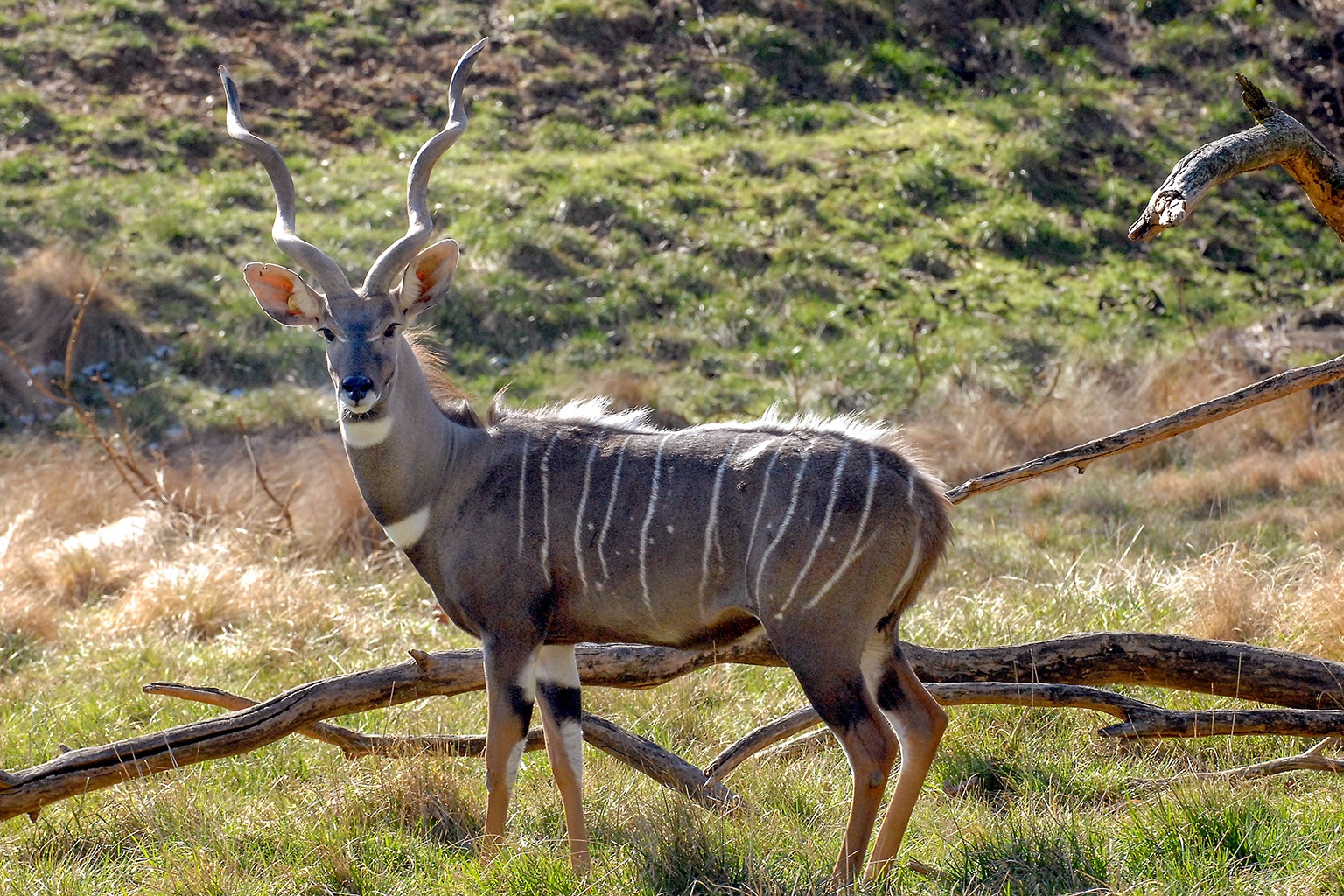This image features an antelope standing in a sunlit meadow, with tall green and brown grass surrounding it and a fallen tree behind. The antelope has striking, tall, and spiraled horns that form an intricate, curly pattern. The horns are nearly three times the height of its head. Its large, erect ears reveal their inner structure, and it directs its gaze toward the camera while its body faces left. The antelope's coat is predominantly brownish-gray, adorned with distinctive white stripes extending from its back to its belly and white patches. The legs display a mix of brown, white, and black, along with some white spots. A furry ridge runs along its back, leading to a curled tail, and the bright sunlight casts sharp shadows and highlights across the scene.